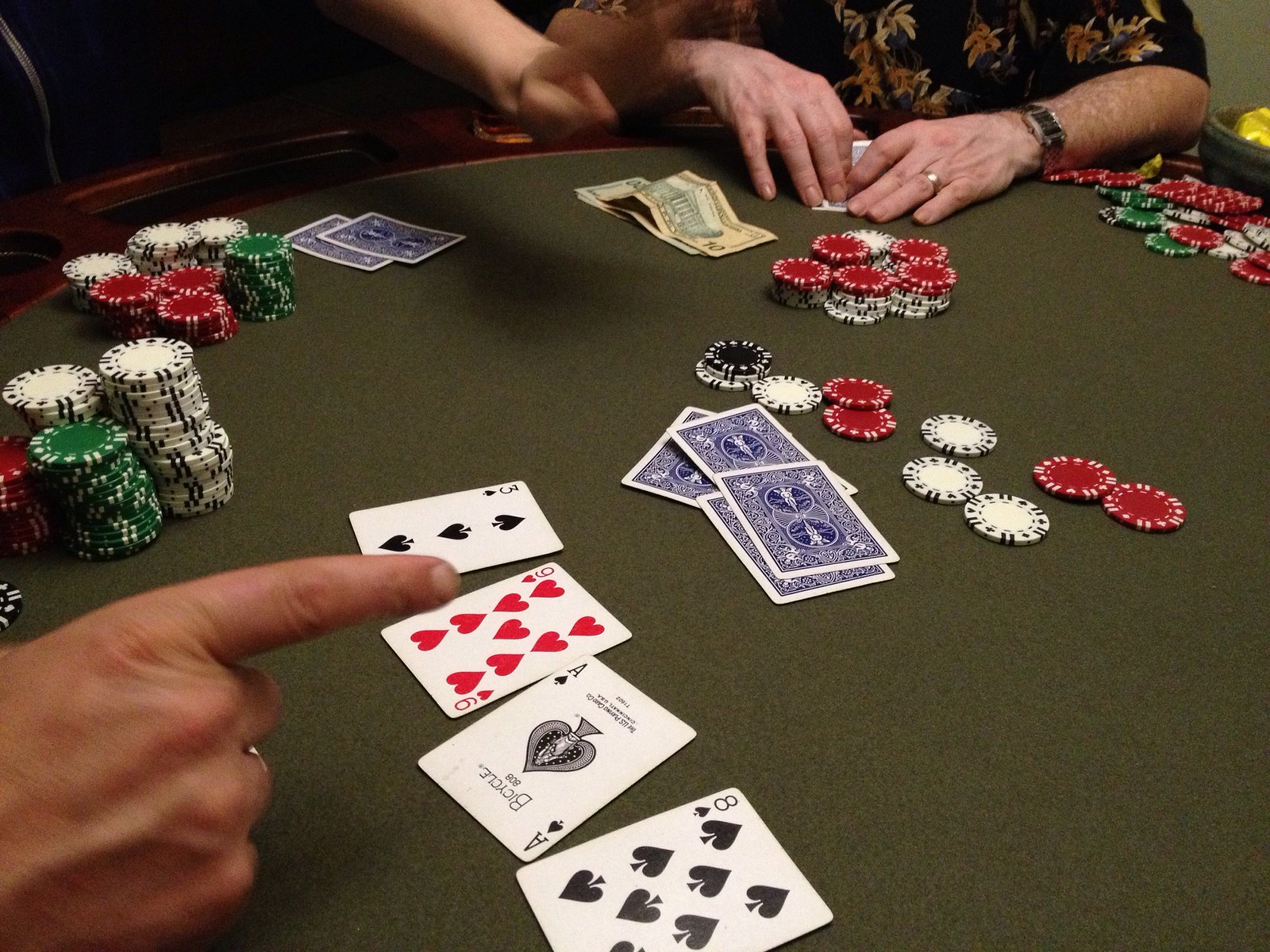The photograph captures an intense poker game in progress, with four pairs of hands giving an insight into the players' strategies. No faces are visible, ensuring the focus remains firmly on the game.

In the foreground, one player is prominently featured, pointing at the table with their index finger. Revealing their hand, four cards are laid out: the nine of hearts, the ace of spades, the eight of spades, and an unclear spade card. A wealth of poker chips, colored in blue, red, and potentially black, are meticulously stacked around the round poker table, with some piles towering higher than others. A smattering of loose chips is also scattered across the table, indicating active play.

Further back, another player is visible at the top of the screen, their hand resting above two face-down cards, suggesting they are awaiting the next move. To the right, another participant has both hands resting on the table, securing one card face down. Beside their hands, there's a $10 bill and two smaller denomination bills, adding a layer of real-world stakes to the game. A cluster of poker chips lies near their arm, which is adorned with a watch, hinting at the passage of time during this engrossing match.